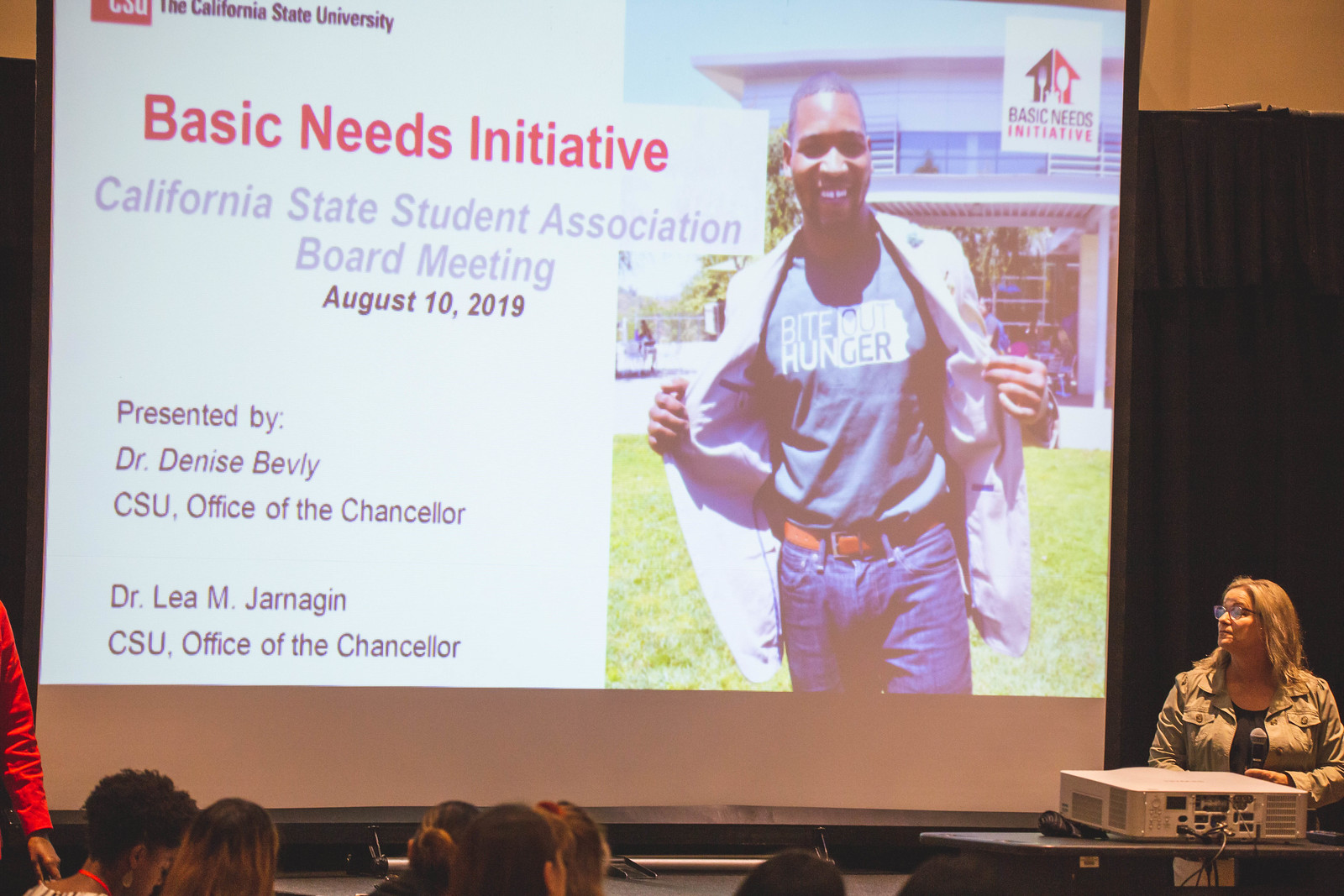The image depicts a presentation at a California State University event, specifically the California State Student Association Board Meeting held on August 10th, 2019. The focus of the meeting is the Basic Needs Initiative, as prominently displayed on a large projection screen on stage. The presentation is being conducted by Dr. Denise Beverly and Dr. Leah M. Jarnagan, both from the CSU Office of the Chancellor. On the bottom right of the image, a woman with golden-colored hair, dressed professionally and wearing glasses, stands near the rotunda. In front of her, there is a table with a computer and other interfaces. Seated at the bottom left of the image are attendees of the presentation, listening attentively.